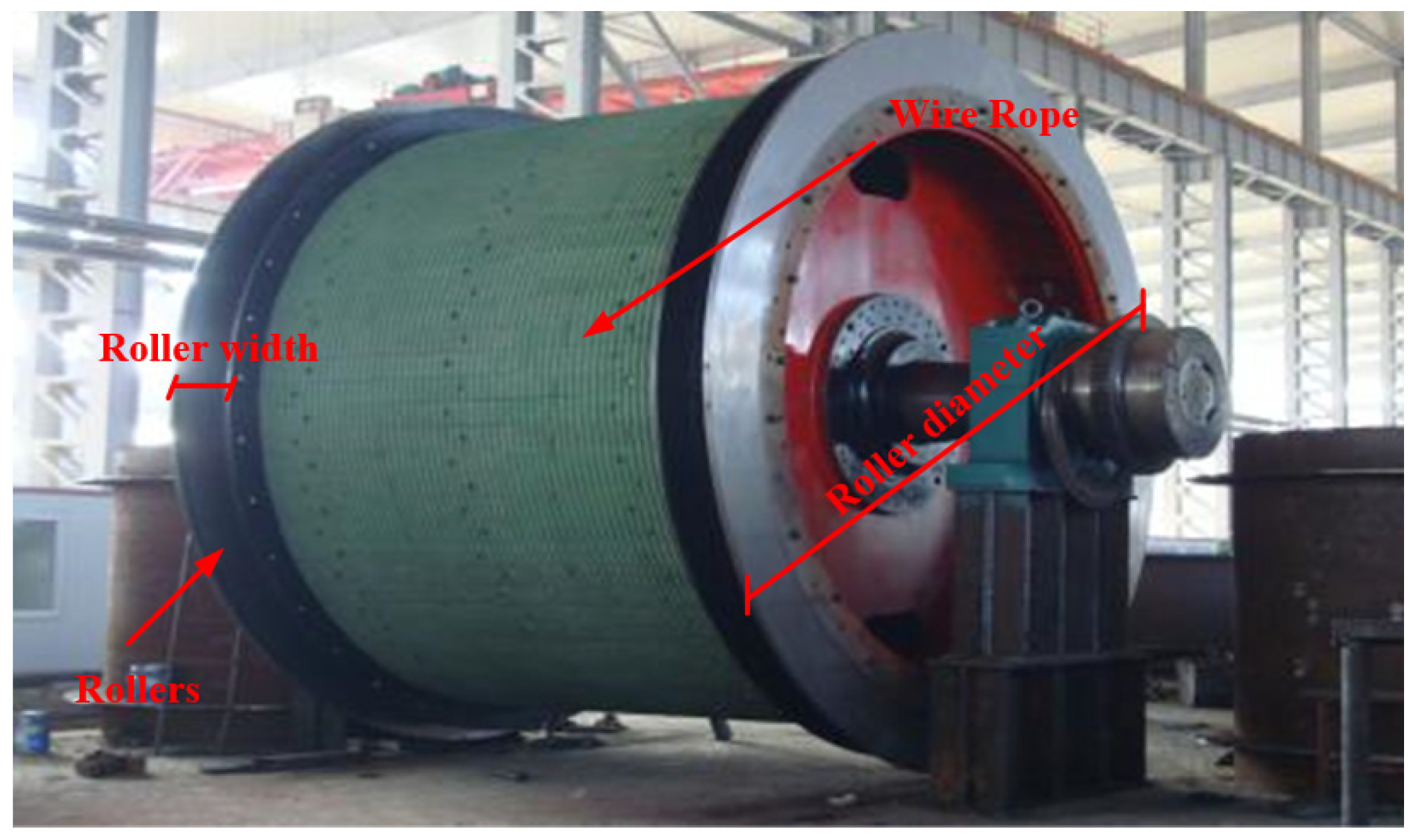The image depicts a large industrial roller located within a vast building featuring prominent iron and steel frameworks, including central girders that support a notably high roof. Illuminated from both the front and back, the photograph shows a significant piece of machinery. The roller is identified prominently by red captions that label various components: "roller," "roller width," "roller diameter," and "wire rope." The roller’s structure includes a red-rimmed, gray shaft that extends to a substantial green metal stand housing a large bearing. The wire rope referred to in the captions is green and wrapped around the roller's circumference, resembling a thick spool of thread. This setup suggests a specialized function, potentially related to mining or heavy-duty industrial processing, as inferred from its size and setting.